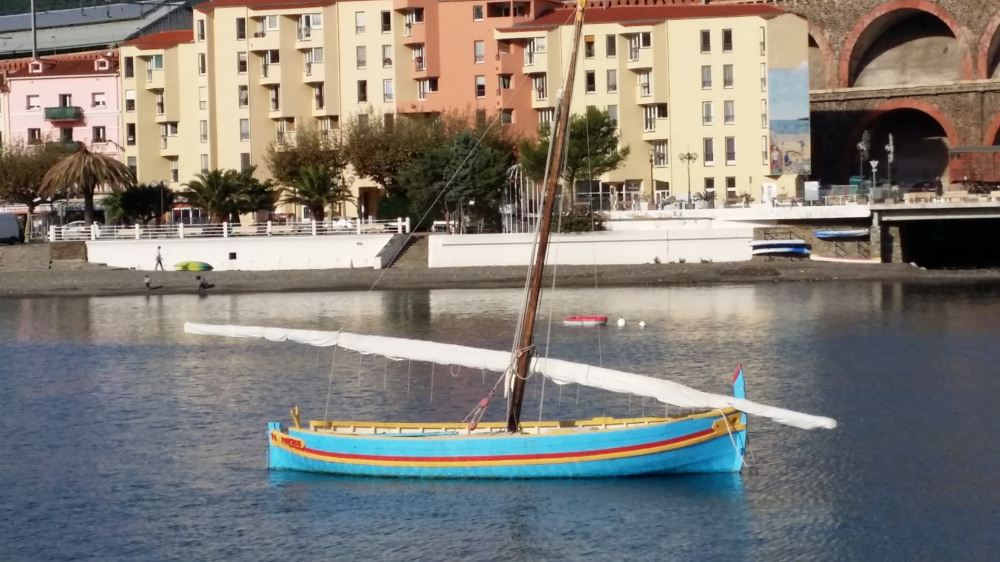The image depicts a picturesque scene of a bright blue, canoe-like sailboat adorned with a red and yellow stripe running from stern to bow. The boat features a wooden mast with a white sail rolled up at its base. Floating serenely in the middle of a tranquil water body, the solitary sailboat is surrounded by a peaceful harbor area. In the distance, you can see the shoreline with a sandy beach adjacent to white-painted steps and railings. A cluster of tall apartment buildings, painted in shades of yellow, red, pink, and cream, lines the shore, some incorporating balconies and many windows. Among the structures, a historic mural and a Roman-style aqueduct or railway bridge with domes add to the scene’s architectural diversity. Adding to the vibrancy, the larger background is dotted with some lush trees, providing a serene contrast to the urban setting. A smaller red and white dinghy can be faintly spotted near the horizon, enhancing the maritime atmosphere of the image.